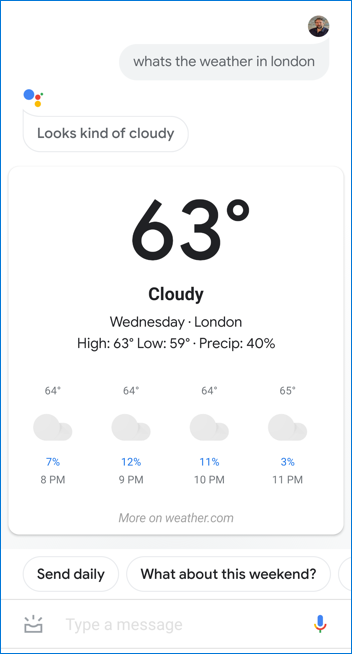The image displays a search results page for the query "What's the weather in London?" in a vertical rectangular format. In the top right corner, there is a round user avatar depicting a young man. Beneath his picture, a gray text bubble contains the query in gray text: "What's the weather in London?" 

To the left, just below this bubble, a blue dot features an icon of a person with a mix of orange and yellow colors. Accompanying this icon is a white text bubble stating, "Looks kind of cloudy." 

The main weather information is presented against a white background. A prominent number "63°" is displayed, indicating the temperature. Below this, bold black text reads "Cloudy," and smaller dark gray text provides the details: "Wednesday, London." Further specifics include "High 63°, Low 59°, Precip: 40%."

Below this data is an hourly forecast represented by four gray cloud icons. The temperatures associated with each hour are: 64° at 8 p.m., 64° at 9 p.m., 64° at 10 p.m., and 65° at 11 p.m. The times are listed directly below, followed by the corresponding precipitation percentages in bright blue text: 7% at 8 p.m., 12% at 9 p.m., 11% at 10 p.m., and 3% at 11 p.m.

Towards the bottom of the image, there are two action buttons. One black text button says "Send daily," and the other asks, "What about the weekend?" At the very bottom, there is a space for typing a message or initiating voice input, indicated by a bright blue and red microphone icon.